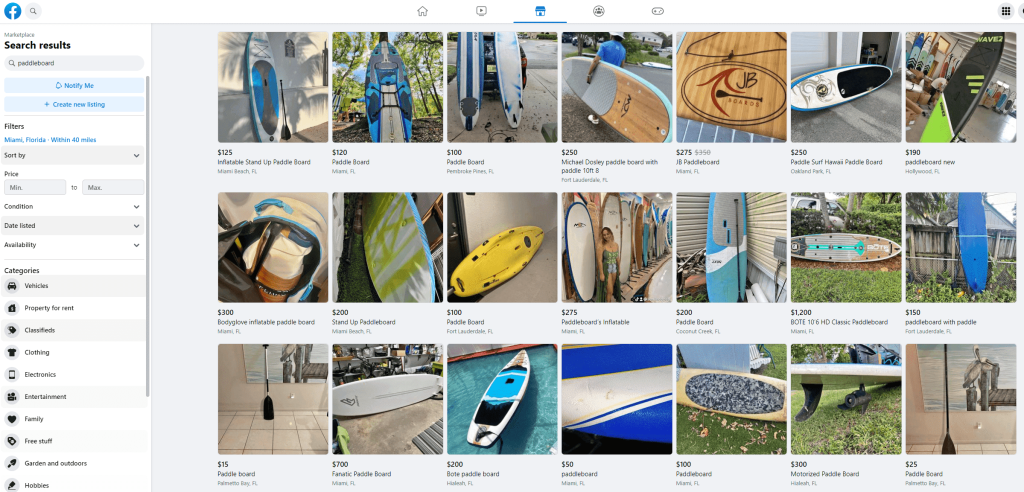The image depicts a desktop screenshot of Facebook, specifically showcasing the Facebook Marketplace interface. The distinct Facebook logo, characterized by a white "F" within a blue circle, is prominently displayed in the top left corner of the screen. Adjacent to the logo is a search icon, followed by icons representing various Facebook functionalities including Home, Facebook Watch, Marketplace (depicted by a little house shop icon), and what appears to be tools for accessing friends lists and notifications.

On the left side of the screen, the search term "paddle boat" is visible, indicating the user's interest. Users have options to be notified of new results or create a new listing. The filters applied include a location set to Miami, Florida, with a search radius of 40 miles. However, no specific sorting criteria have been selected. Additional filter options are visible, such as price range (minimum to maximum), condition, date listed, and availability.

Below these filter options, the various categories within Facebook Marketplace are displayed, including vehicles, properties for rent, classifieds, clothing, electronics, entertainment, family, free stuff, gardens, outdoors, and hobbies. Each category is represented by small icons like a car, house, price tag, shirt, phone, video camera, heart, book, shovel, and art pen.

On the right side of the screen, there are 15 search results showing a variety of paddle boats available within the specified area. The listings range in price from $15 for a basic paddle board to $300 for more expensive options. The paddle boards come in various colors but generally maintain the same shape and design.

In summary, the screenshot highlights Facebook Marketplace search results for paddle boards within 40 miles of Miami, Florida, illustrating the diverse options and price ranges available to potential buyers.